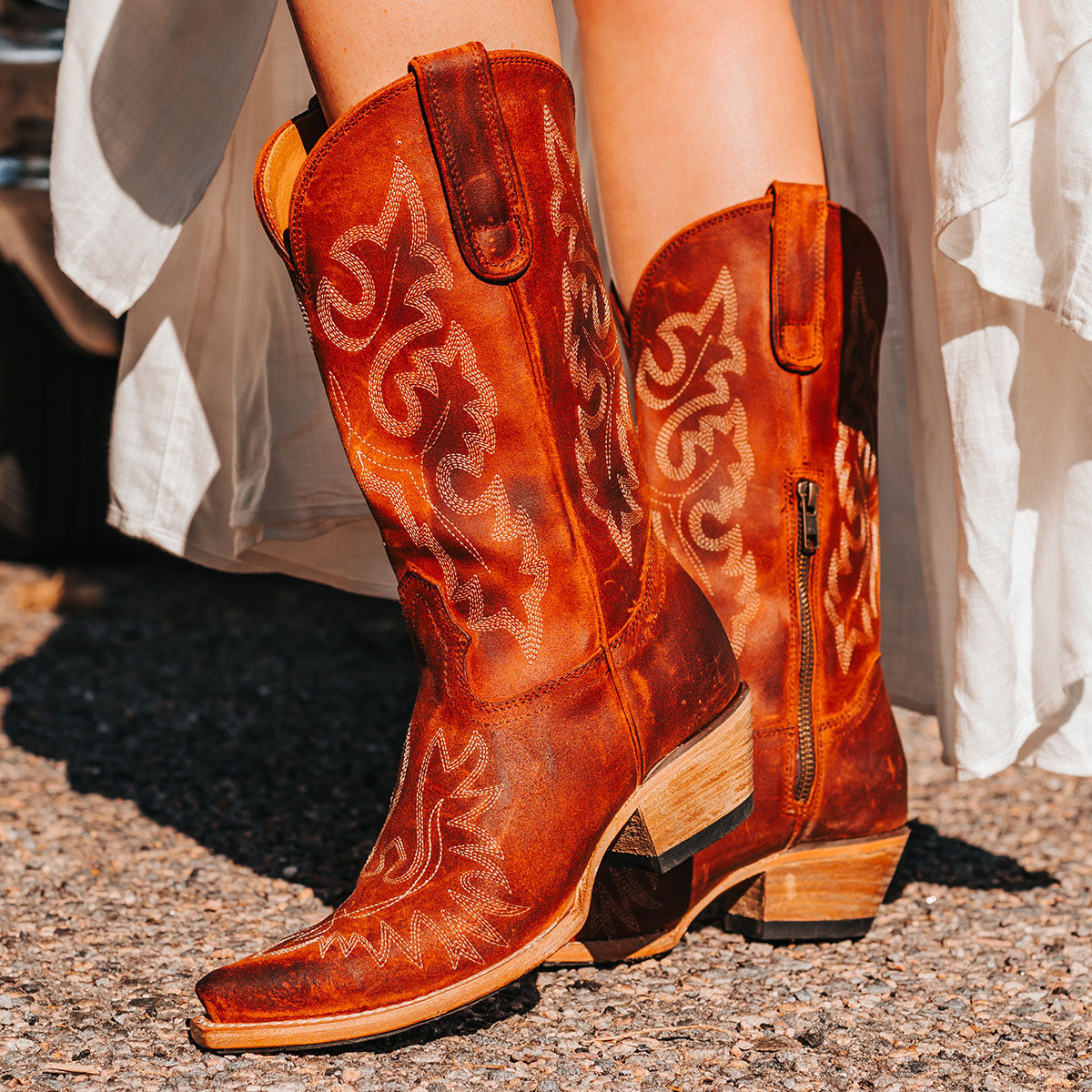In this detailed image, a young woman is showcasing her stylish, rich brown leather cowboy boots against a backdrop of brown gravel. She is dressed in a long, flowing garment—possibly a white dress or coat—that billows down to her calves. The garment is held up slightly to reveal her smooth Caucasian legs and the boots, which stand out as the focal point of the photo. The cowboy boots feature intricate white stitching on the sides and top that resemble leaf patterns. One foot is positioned flat on the ground, while the other is lifted slightly. The boots have a sturdy wooden sole and a modest heel, estimated to be between one to two inches high, providing a slight lift. Notably, there is a small zipper on the outside of one boot, likely serving as a decorative element rather than a fastening mechanism. The photo captures the rugged elegance of the boots, emphasizing their craftsmanship and the contrast between the delicate fabric and the tough terrain.